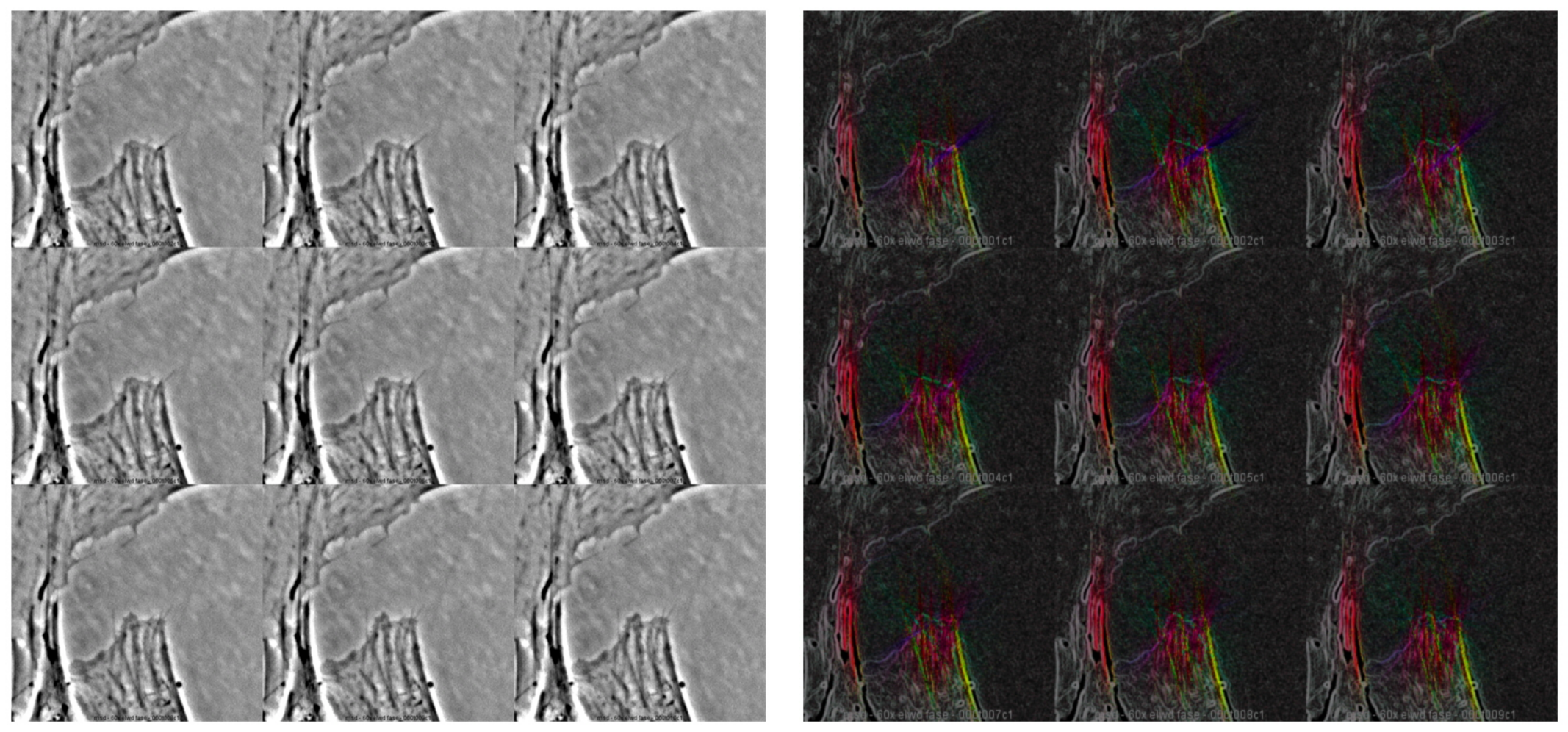The image features two artworks presented side by side, each composed of nine blocks arranged in three rows and three columns. The artwork on the left has a monochromatic gray palette with intricate, stone-like engravings forming geometric designs that resemble tents or teepees. This left-hand image is uniform in color, utilizing various shades of gray to create a textured effect. In contrast, the artwork on the right shares the same nine-block layout and design, but features a stark black background. The geometric shapes in this version are vibrant, with colors including red, yellow-green, light gray, and hints of purple. These colors give the impression of dynamic, possibly volcanic, activity, providing a vivid contrast to the subdued tones of the left artwork.